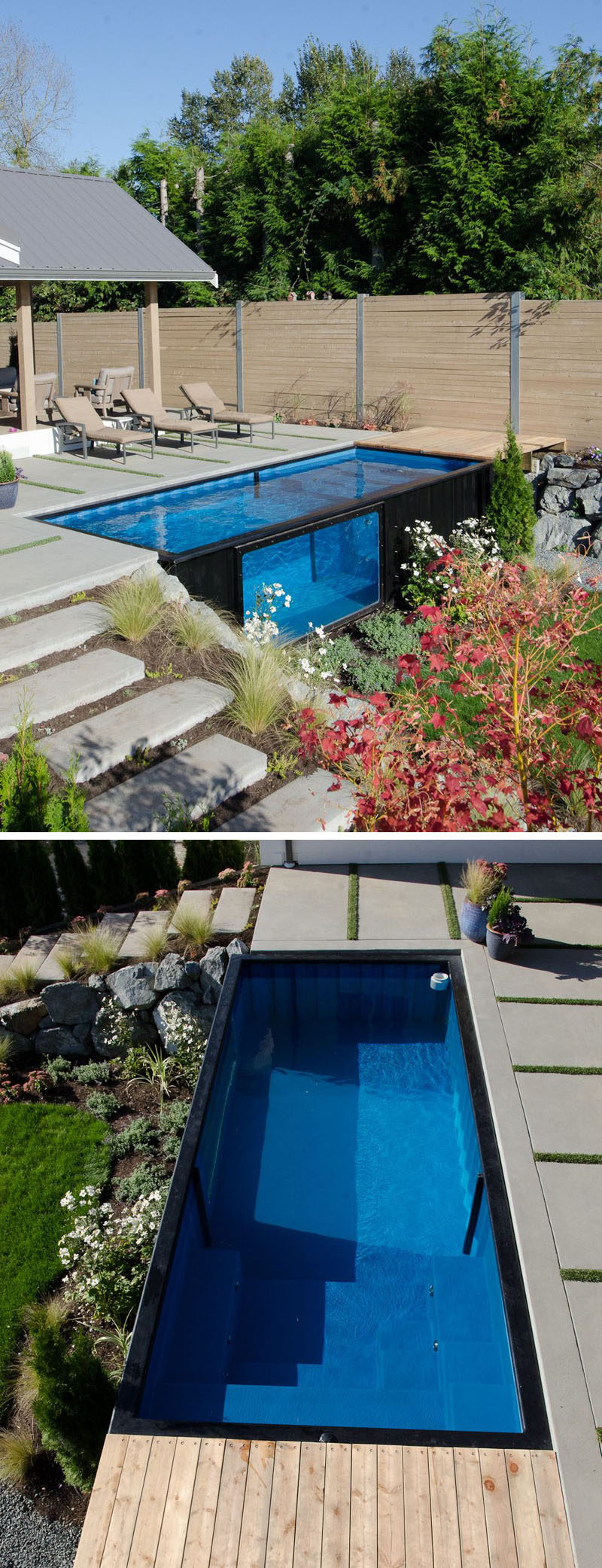The image consists of two vertically stacked photographs showcasing a stunning outdoor saltwater pool area during daytime. In the top photograph, against a backdrop of clear blue sky and green trees, a rectangular infinity pool is featured with a glass side panel, resembling a window into the pool. The pool is surrounded by a concrete deck accented with thin bands of grass and features three lounge chairs arranged to overlook the pool. The surrounding landscape includes carefully manicured greenery and a privacy fence. Stone steps to the left lead down to the pool area, while a covered patio behind the pool hosts additional lounging furniture. On the right side, a shrub with light pink flowers adds a touch of color.

The bottom photograph offers a closer look at the serene pool from a different perspective, highlighting the pool's deep blue water bordered by a sleek black outline. More of the meticulously landscaped area is visible, including the grassy patches and the stone steps seen at the top of the image. In the top right corner of this photo, three cactus pots are arranged on the deck. The pool area is further complemented by a partial wooden deck with thin horizontal stripes. Overall, the scene captures the elegance and tranquility of this well-designed outdoor oasis.